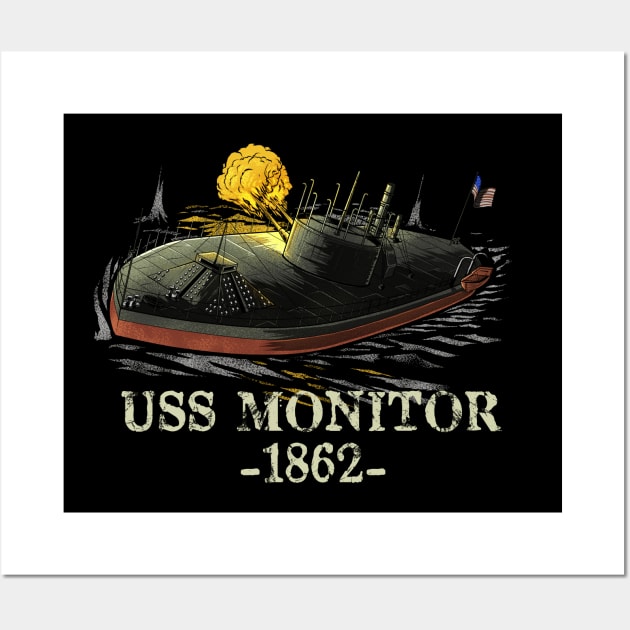The photograph depicts a framed piece of wall art hanging on a greyish-white wall, enhanced by a slight drop shadow. The artwork features a battle scene centered around the historic ship, the USS Monitor, as indicated by the white text at the bottom which reads "USS Monitor 1862" with an aged, scratched effect. The art itself is square-shaped with a white border and a stark black background. In the center, a large ship—stylized as a battleship or submarine—is shown in the midst of combat, firing from two prominent cannons on its left side, while a yellow explosion erupts at the top. The deck of the ship is grey, while its hull is painted a bold red. The black-colored sea beneath the ship is accentuated with grey stripes. Completing the scene, a United States flag flutters in the upper right corner, contributing to the vivid narrative of historic naval warfare.